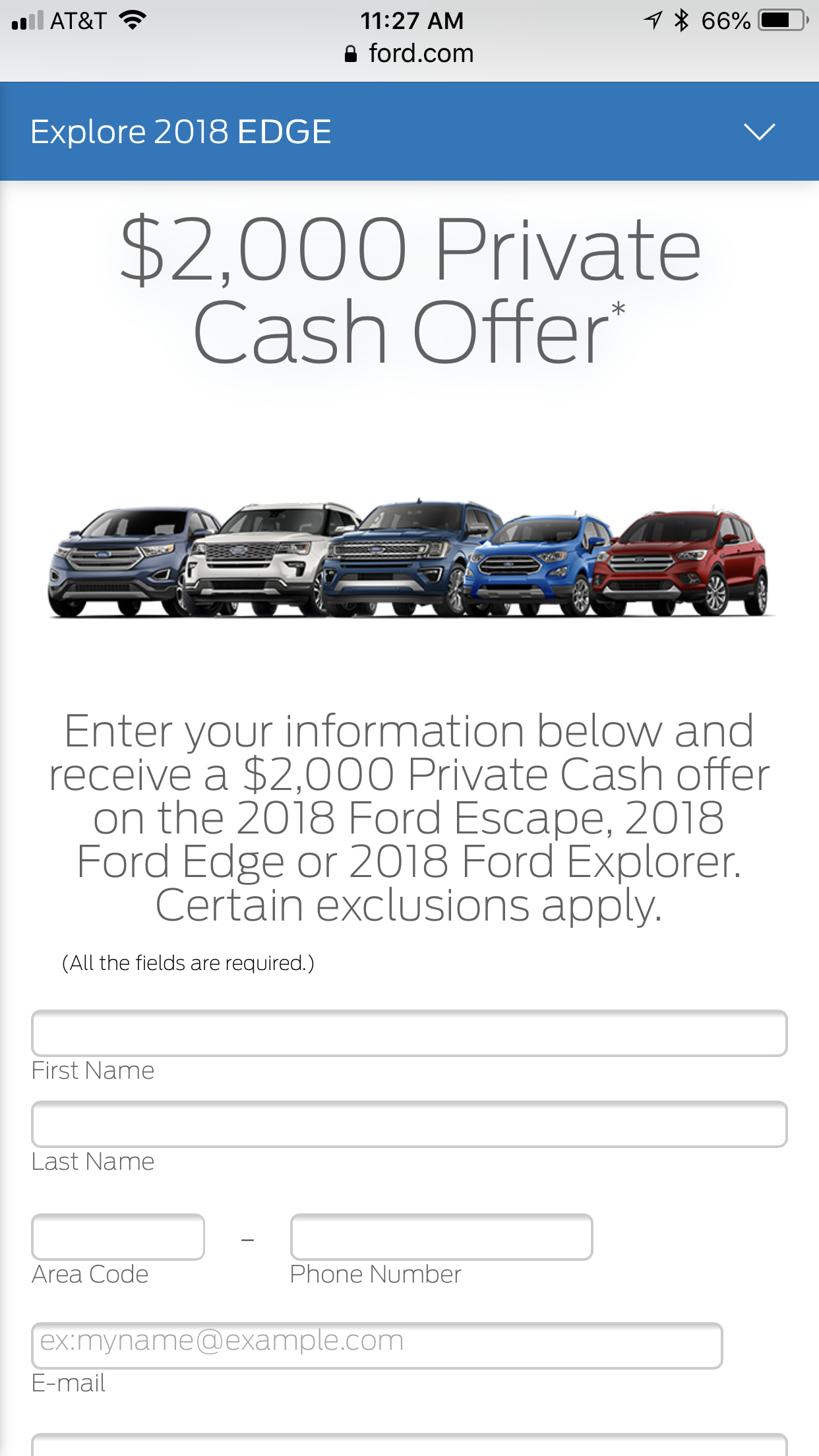The image is a screenshot from a website, captured on a device displaying a light gray banner at the top. The banner includes various status indicators such as the cellular signal showing "AT&T," a Wi-Fi signal, and the current time indicated as "11:27 AM" in black text. Next to the time, there's a padlock icon, accompanied by the text "ford.com," indicating a secure connection. On the right, there are symbols for Bluetooth connectivity and battery status, which shows 66% remaining.

Below this gray banner, a blue banner runs across the width of the screen. On the left side of this banner, the text "Explore 2018 EDGE" is displayed in capital letters, with a downward-pointing arrow on the right, suggesting a dropdown menu.

The main content of the page is set against a white background, featuring a headline in bold font: "$2,000 Private Cash Offer," marked with an asterisk. Below this headline, there are pictures of five vehicles, categorized as SUVs, smaller SUVs, and cars. The accompanying text reads: "Enter your information below and receive a $2,000 Private Cash Offer on the 2018 Ford Escape, 2018 Ford Edge, or 2018 Ford Explorer. Certain exclusions apply." 

In smaller print, a note indicates: "(All fields are required)." The form below this note includes blank spaces for "First Name," "Last Name," "Area Code" followed by a hyphen, "Phone Number," and "Email." The final input field is partially cut off, making it unclear what information is being requested.